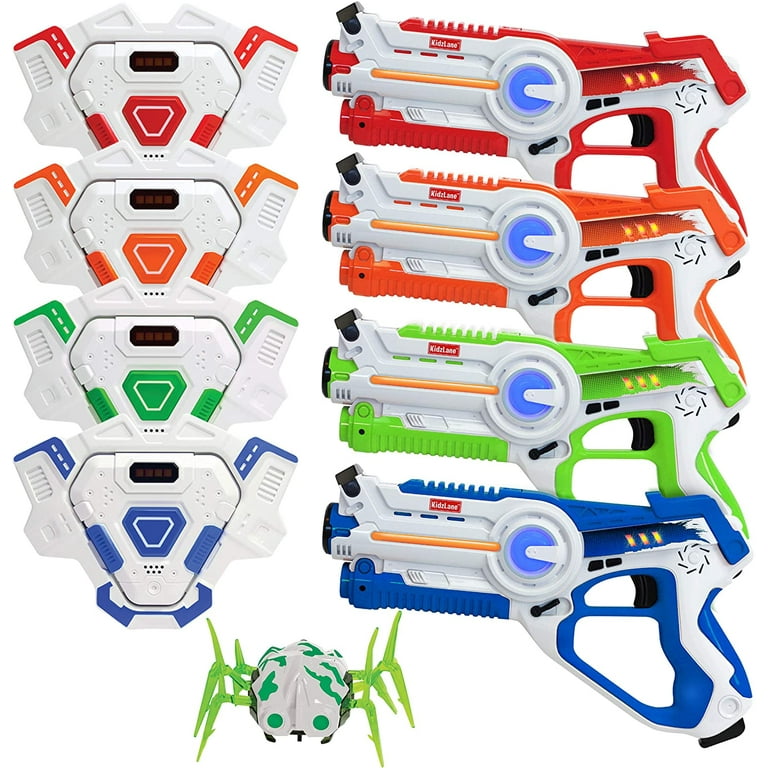The image features a collection of colorful toy guns and triangular-shaped objects arranged on a white background. There are two vertical columns of toys: on the left, the toys are white with accents in red, orange, green, and blue from top to bottom, each resembling a remote control with additional handles extending like wings. On the right, right-facing toy guns correspond to the colors of the left-side objects, following the same red, orange, green, and blue color scheme from top to bottom. Positioned at the bottom center of the image is a spider-shaped toy, white with green spots and pale green legs, facing outward with striking green eyes.